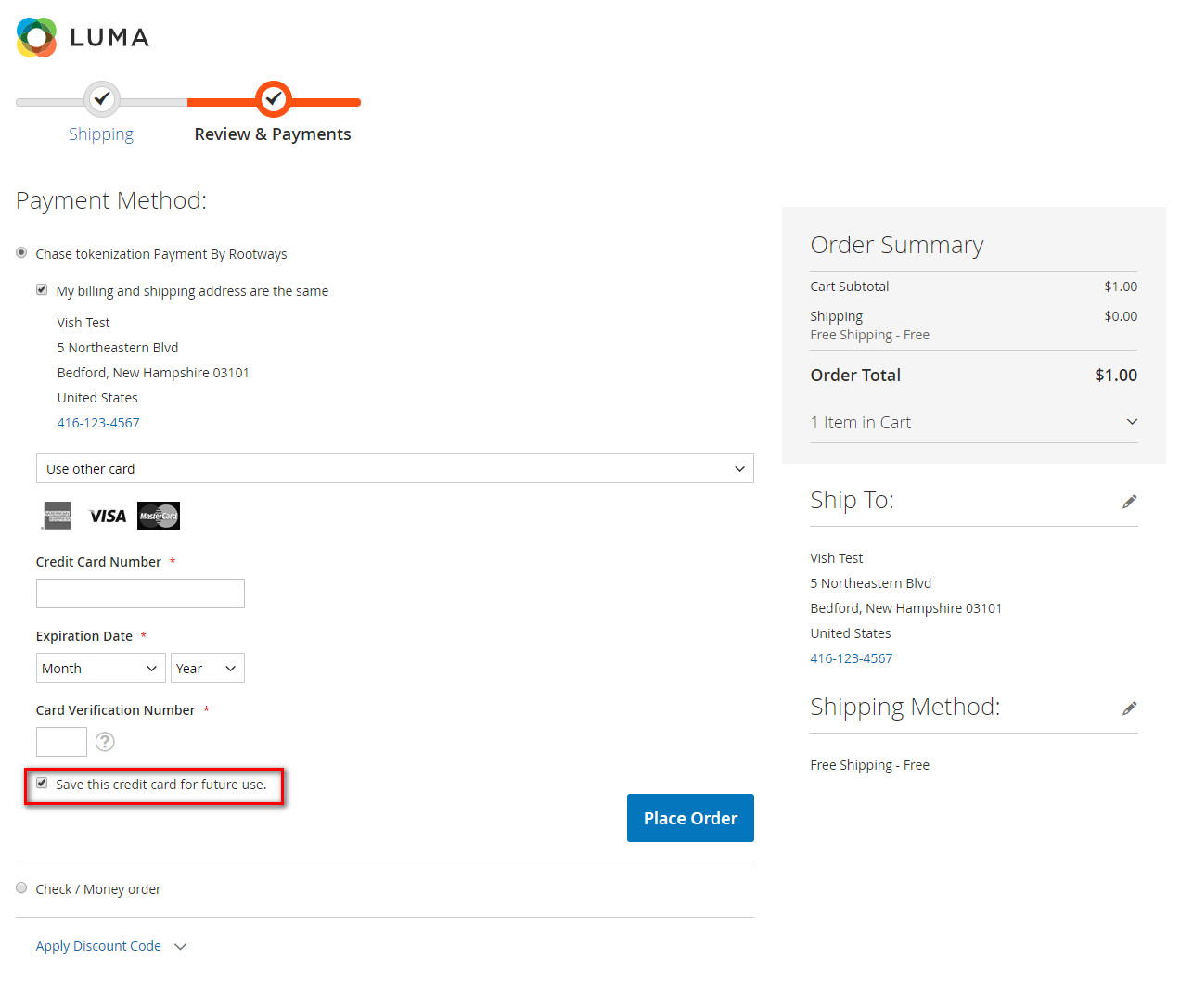In the image, we see an order window set against a pristine white background. At the top of the window, the brand name "Luma" is prominently displayed, accompanied by a circular logo reminiscent of a Simon Says game, segmented into blue, green, yellow, and red sections. Below the logo, navigation options are presented: Shipping and Review Payments, with the latter highlighted in orange, indicating the current page.

The main section outlines the payment method, specifying "Chase Tokenization Payment by Rootways." It also includes an option to confirm that the billing and shipping addresses are the same, displaying the address: Vishtas, 5 Northeastern Boulevard, Bedford, New Hampshire, 03101, United States, and the phone number 416-123-4567. Further down, there's a section for using credit cards, featuring logos of Visa, MasterCard, and American Express, along with fields to enter the credit card number, expiration date, card verification number, and an option to save the card for future use.

On the right side of the window, there is an order summary breaking down the costs: Cart Subtotal of $1, Shipping at $0, leading to an Order Total of $1. The shipping address is reiterated: Vishtas, 5 Northeastern Boulevard, alongside the note that the shipping method is free. Additionally, there is a blue "Place Order" button, ready for the final step of the transaction. Lastly, an "Apply Discount Code" section is available for users to enter any promotional codes they might have.